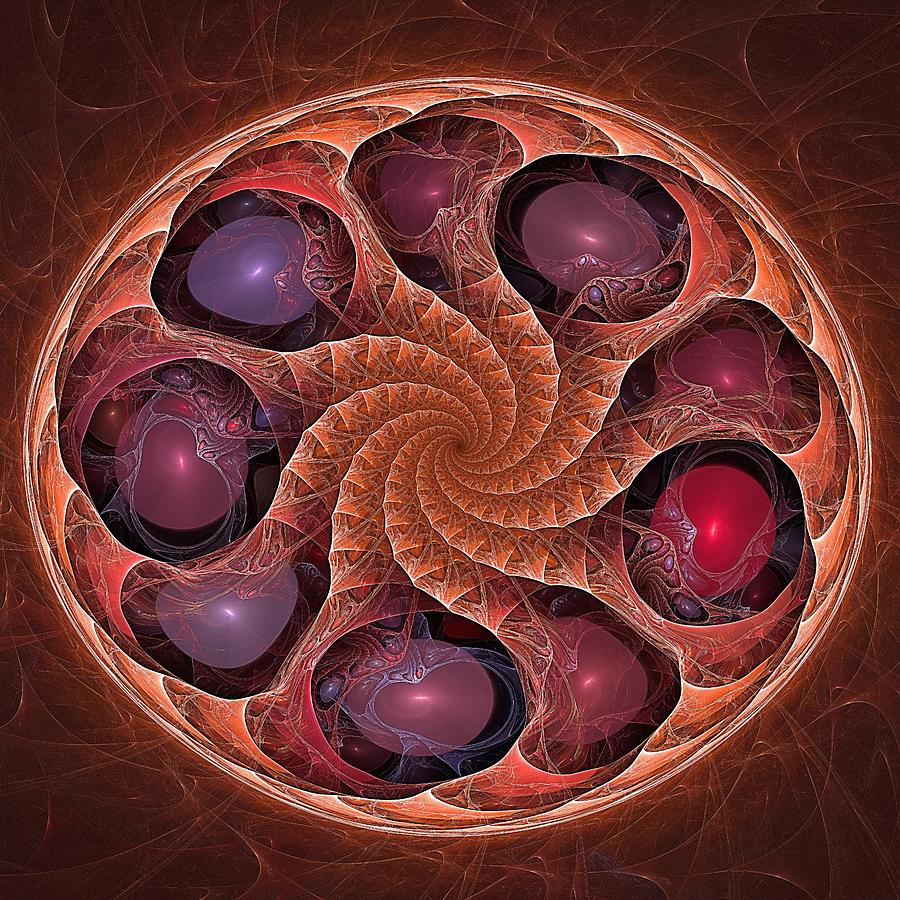This image is a highly detailed and abstract computer-generated illustration featuring a central spiral pattern reminiscent of a seashell or coiled membrane. At the core of this spiral are nine reflective, jelly bean-like eggs or balls in varying shades of purple—from dark purplish-red to light purple and purple-blue. Arranged in a subtle clockwise rotation, these eggs are embedded within a spiral backdrop that curves gracefully at specific intervals, somewhat like segmented lobster tail scales.

The entire composition is enveloped in a dark red background interspersed with transparent, spiderweb-like layers, adding a sense of depth and complexity. Light reflections on the surface of the eggs and the spiral itself lend a 3D effect, making the scene look almost otherworldly and sci-fi-esque. A white, circular border surrounds the entire image, which is further accentuated by larger scales that seem to encroach from the edges, giving an impression of containment within a membrane. The overall ambiance is both intriguing and slightly unsettling, akin to a surreal, biological structure magnified under a microscope.